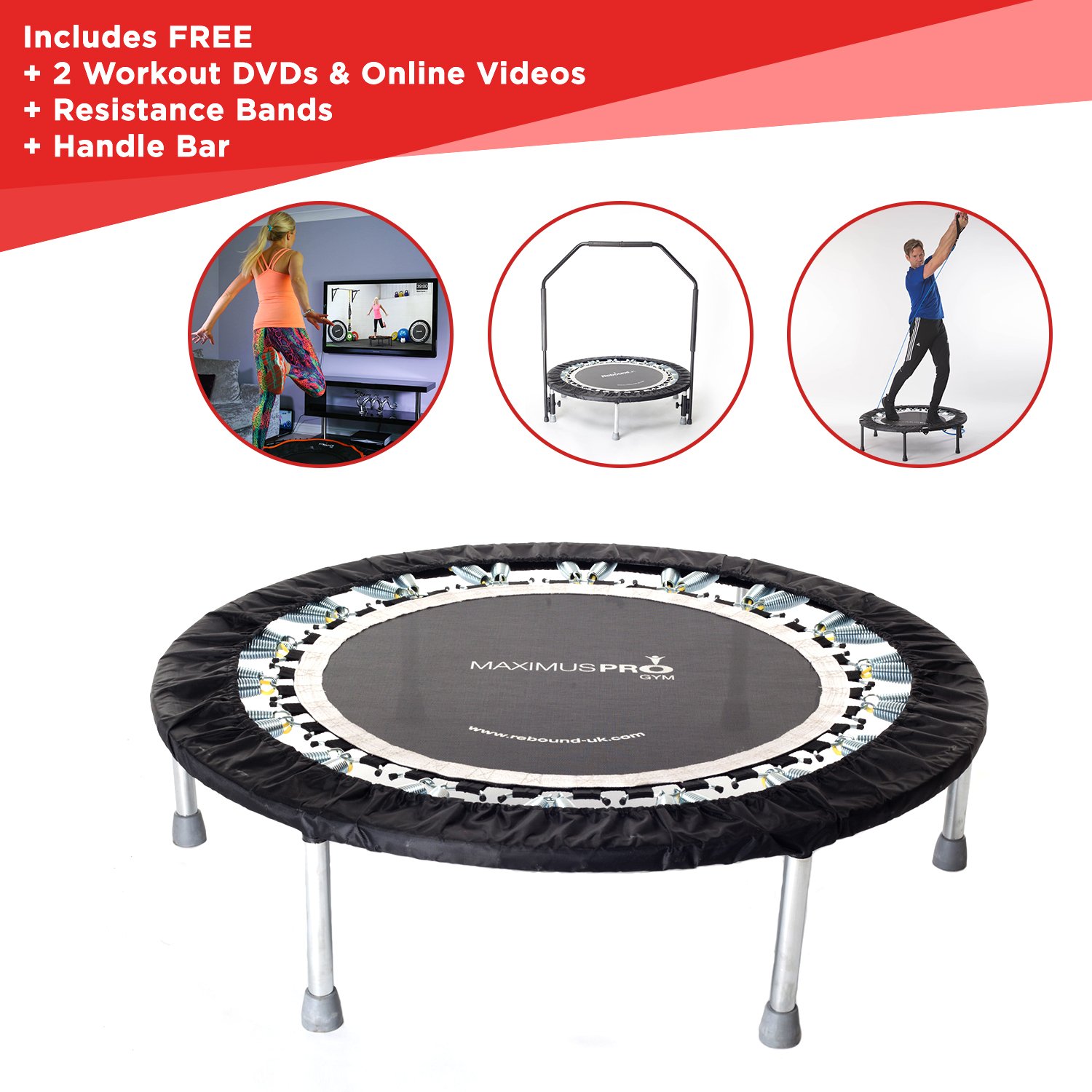The image is an advertisement for a small personal trampoline. The main focus is the close-up view of the trampoline situated at the bottom center, showcasing its detailed features. The trampoline is black, with a white ring around its edge and silver springs connecting it to a black cover. It stands on six silver legs with gray feet. Above the trampoline, there are three small red-circled photos, each depicting different uses of the trampoline. The left photo shows a woman jumping and working out to a video in a blue room. The center photo highlights a version of the trampoline with an arch attachment. The right photo features a man using pulley exercise equipment while on the trampoline. At the top left, a red banner with white text advertises, "Includes free: two workout DVDs and online videos, plus resistance bands, plus handlebar." The image collectively presents the trampoline's multiple functionalities and extras included in the offer.